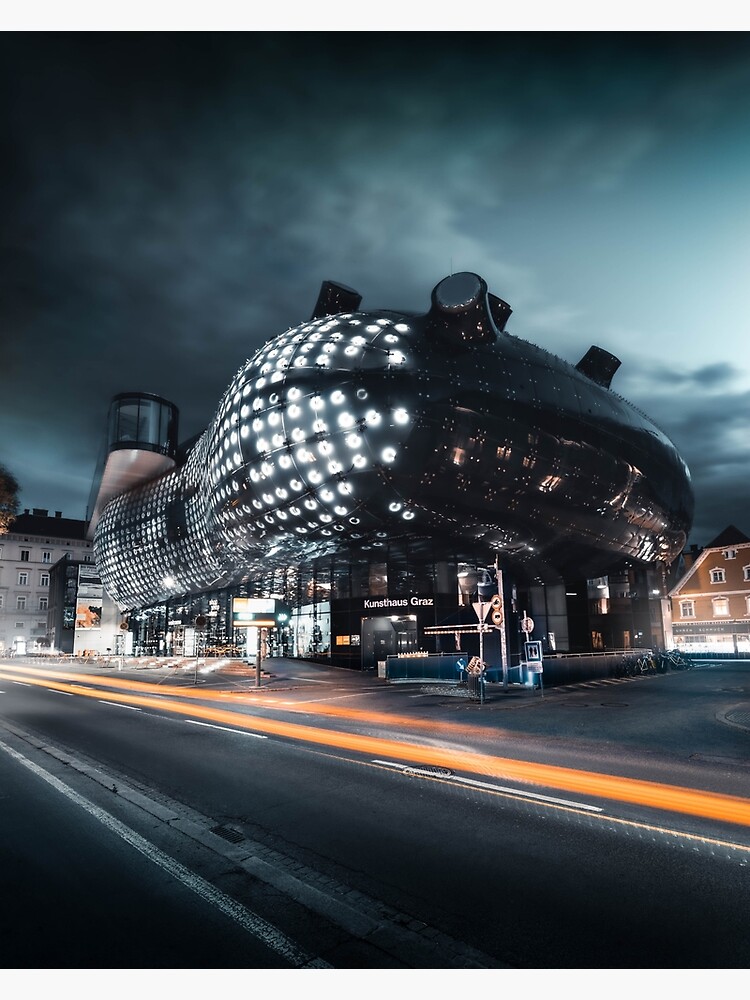In the center of a dark, futuristic cityscape looms an imposing, spaceship-like building labeled "Kunsthaus Graz." This otherworldly structure, with its sleek, chrome exterior and illuminated nodules on top, stands out against the inky black sky filled with dark clouds. A highway, starkly empty of cars, runs along the bottom of the image, with one side painted orange. The scene is completely devoid of people, adding to the eerie, surreal ambiance. Despite its late-hour setting—whether evening or early dawn—the building emanates a mysterious glow from its various circular light sources and internal lights. Traditional European-style apartment buildings are visible in the background, enhancing the contrast with the ultra-modern, almost alien appearance of the Kunsthaus Graz. The photo, likely touched-up or photoshopped, captures a moment of quiet solitude in a metropolitan environment, with the street framing the bottom of the picture, mostly on the left side.